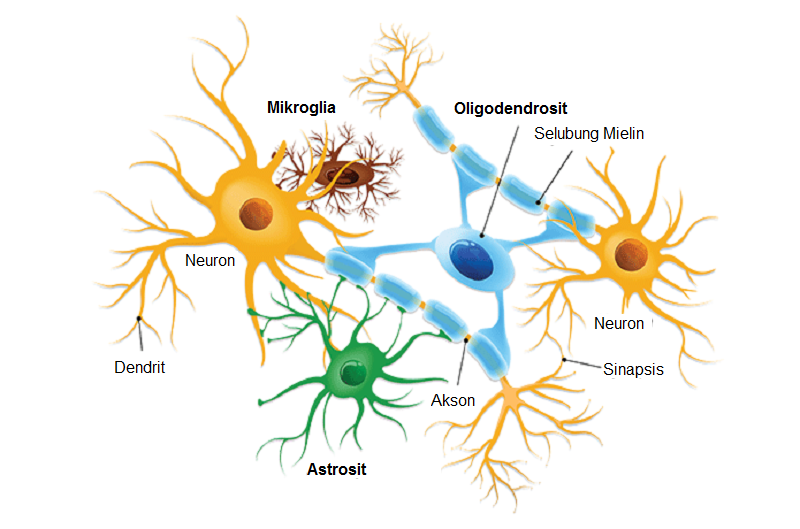This detailed scientific illustration on a white background depicts various types of brain cells and their components, color-coded for clarity. At the forefront are yellow neurons, characterized by their branched tentacles. The text labels "neuron" and "axon" highlight the neuron’s connection to the blue-labeled "oligodendrocyte" cells and the blue "myelin" sheath. Brown microglia and green astrocytes, each with branching structures, are also identified. Additional text on the diagram includes synapses, dendrites, and Celebung myelin, providing a comprehensive overview seen in educational materials like school or university textbooks. The illustration’s intricate details and text annotations suggest its purpose for learning and understanding neural biology.